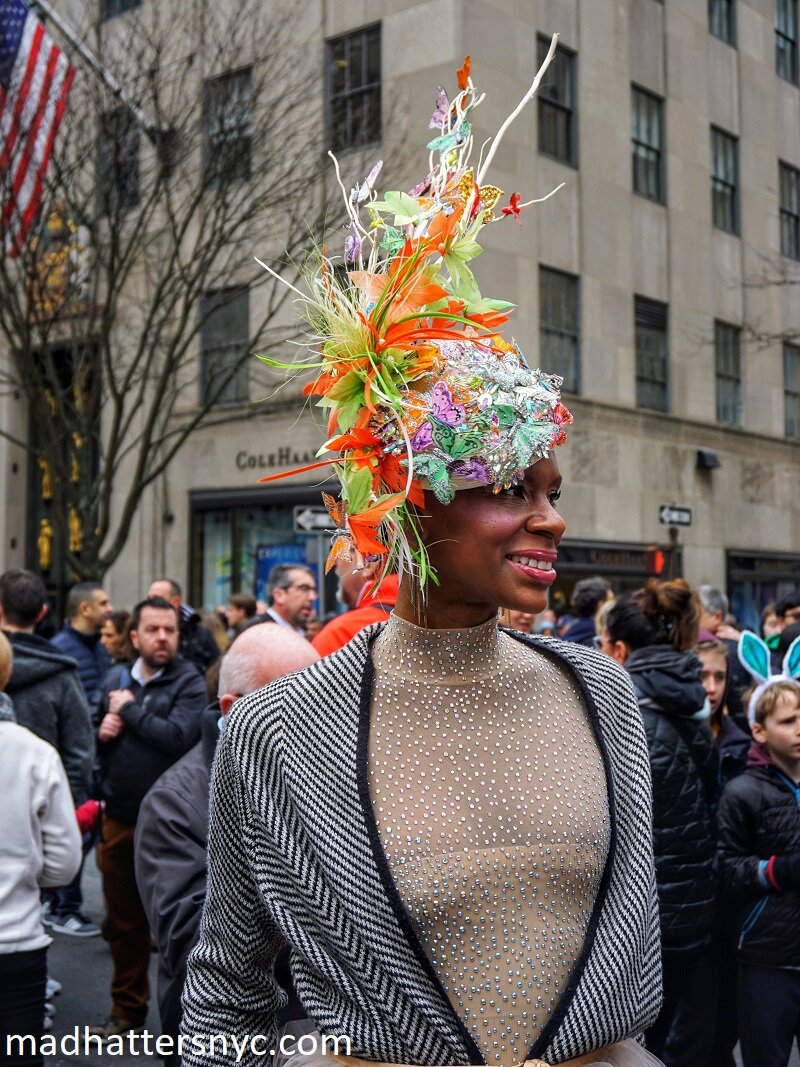In a bustling city street, likely New York City given the watermark "MadHattersNYC.com," stands an elegant and slender African woman who draws immediate attention. She wears a striking, semi-transparent beige turtleneck adorned with shimmering details, paired with a zebra-striped cardigan. Her head is adorned with a spectacular and colorful hat featuring an array of flowers in green, orange, light purple, and white, as well as butterflies and glittering sequins, with tendrils of flowers extending upward. Her bright red lipstick and radiant smile further accentuate her vibrant presence as she gazes off into the distance.

The scene suggests a festive gathering, potentially an Easter event, inferred from the child in blue and white bunny ears visible to the right of the image, amidst a diverse crowd of men, women, and children of various races and ages. In the background, an American flag hangs from a building identified by letters spelling "COLEHAAL," adding to the urban setting. The bare tree in the foreground hints at the possibility of it being autumn or winter, contrasting with the vivid energy of the hat-wearing revelers around her. A "One Way" street sign and the presence of the American flag subtly detail the city atmosphere, completing this lively and colorful urban tableau.